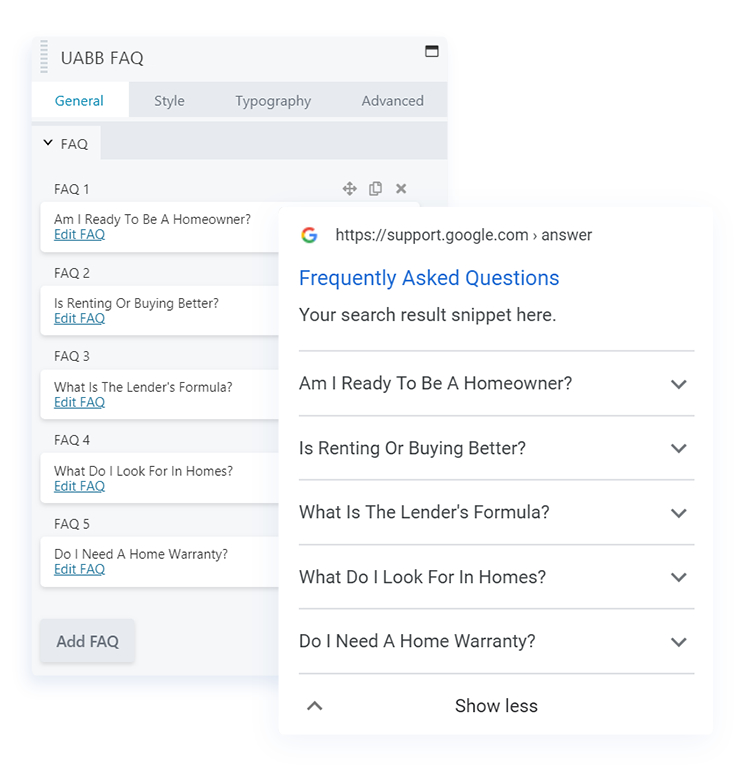The image showcases a screenshot set against a white background, featuring two distinct screens. 

On the left side of the screenshot, there is a user interface section with a light blue background labeled "UABB FAQ" in dark blueprint. This section displays a series of tabs along the top, from left to right: General, Style, Typography, and Advanced. The 'General' tab is highlighted in white, suggesting it is currently active. Below this, a list of FAQs is presented: 
1. "Am I ready to be a homeowner?"
2. "Is renting or buying better?"
3. "What is the lender's formula?"
4. "What do I look for in a home?"
5. "Do I need a home warranty?"

There is also an 'Edit FAQ' link and a prominent blue button labeled "Add FAQ" situated below the list.

To the right of this section, an open webpage is visible with a 'G' icon in the upper left corner, indicating it is a Google support page. The webpage URL is "support.google.com/answer" and features a heading in blue text titled "Frequently Asked Questions." Below this heading is a placeholder for search results, which currently displays, "Your search results snippet here." The first FAQ, "Am I ready to be a homeowner?" includes a pull-down arrow next to it, indicating additional information can be expanded.

Overall, the image captures an interface for managing Frequently Asked Questions alongside a Google support page, providing a comprehensive view of how FAQs can be edited and displayed.